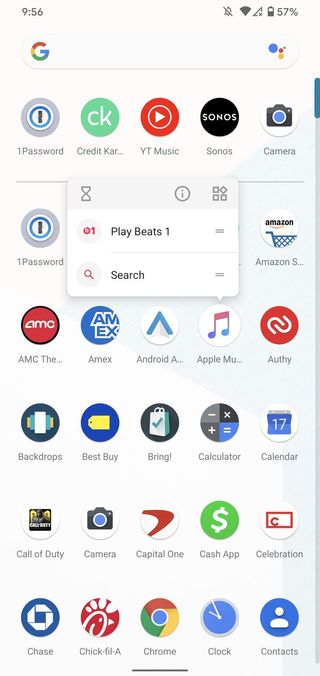This is a detailed screenshot captured on an Android device, displaying the app drawer with all the installed applications arranged in alphabetical order. At the top of the screen, numerical apps are listed first, followed by apps starting from the letter A and proceeding to Z. The first row showcases frequently used or suggested apps, which include "1Password," "Credit Card," "YouTube Music," "Sonos," and "Camera." 

Below this row, there are interactable elements such as a "Play Beats 1" button and a "Search" bar for easy navigation. The diverse collection of apps on this device continues with titles like "Call of Duty," "Camera," "Capital One," "Cash App," "Celebration," and others. Further notable apps include "Contacts," "Chick-fil-A," "Chase," "Calendar," "Calculator," "Best Buy," "Backdrops," "Amex," and native apps like "Android." This screenshot provides a comprehensive view of the individual’s app ecosystem, reflecting varied interests and utilities.